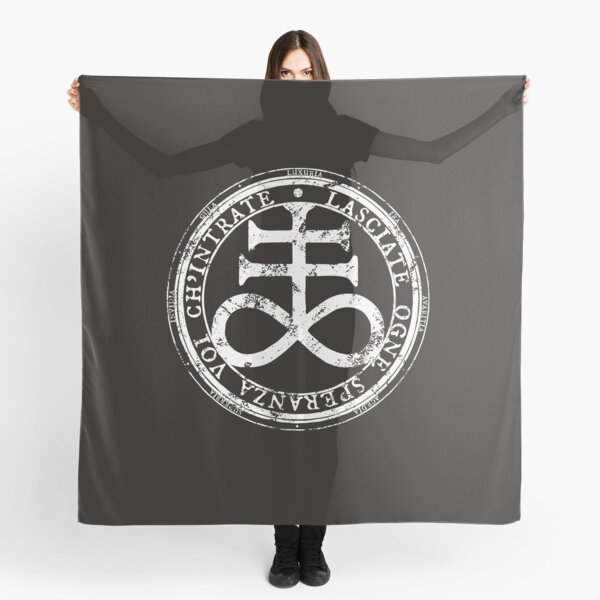The photograph portrays a woman standing against a solid white background, holding a large, translucent black tapestry. The tapestry is so sizeable that it conceals most of her body, with only her eyes peeking over the top and her black shoes visible at the bottom. Her straight, dark brown hair is parted in the center, and her arms, wearing a short-sleeved shirt, are extended to grasp the edges of the tapestry, allowing parts of her silhouette to show through. 

The tapestry itself features a distinctive insignia in the center: a white Celtic cross with a double crossbar atop an infinity symbol, all surrounded by a series of concentric circles and inscribed with white text in a foreign language, possibly Latin or Irish. The text around the circles include the phrase, "CH'apostrophe intrate lasciate agni speranza," and the word "Lingerie" is also discernible among the tiny texts within the outer ring.